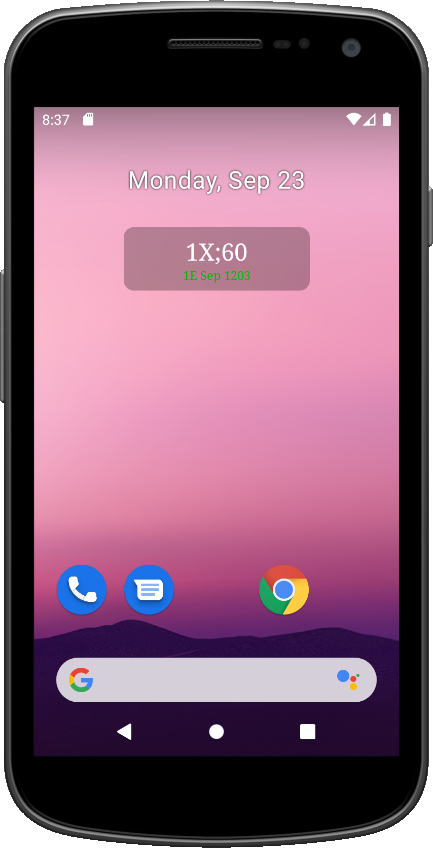The image features a modern cell phone, reminiscent of an iPhone, with a sleek silver frame. The back of the phone is black at the top, sides, and bottom. The screen displays a gradient background transitioning from light pink at the top to dark pink, then to purple at the bottom, with a mountain range image.

At the top of the screen, the time is displayed as "8:37." To the right, icons show the SIM card status, Wi-Fi signal, cellular signal strength, and battery life. Beneath the time, the date is displayed as "Monday, SEP 23."

In the center of the screen, there is a rectangular widget with curved edges displaying "1X; 60" in lime green, followed by "1E SEP SEP" and the time "12:03" below it.

At the bottom of the screen, there are three blue circular icons. The first contains a white phone, the second shows a white speech bubble with lines representing text, and the third is a circle for the Google browser. A search bar, marked with the letter 'G,' sits at the bottom of the screen. Below the search bar, navigation icons feature a left-facing arrow, a circle, and a square, positioned from left to right.